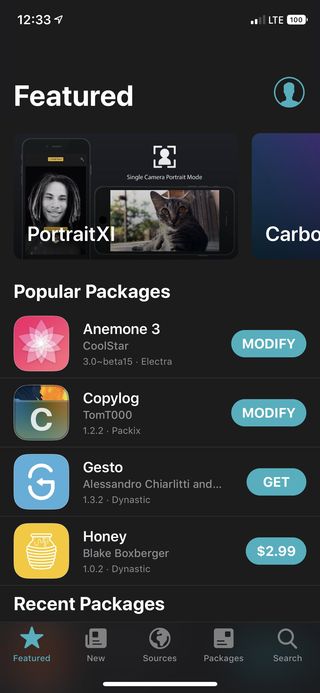A detailed description of the smartphone screen image:

The smartphone screen displays the time as 12:33, located at the top left corner. The device is connected to LTE and has a full battery life indicated by the 100% battery icon. The screen has a dark background, and at the top, 'Featured' is displayed in white text. Below that, there is a silhouette of a profile picture in blue.

The lower part of the screen features sections labeled 'Portrait XI' showcasing a smartphone with an image of a face on it. Adjacent to it is another section labeled 'Single Camera Portrait Mode' displaying a portrait of a cat. Below these sections is a list of popular packages.

One of the packages listed is 'Anomane 3 by Coolstar,' marked with version '3.0 beta 15 electrica,' and it has a 'Modify' button. Another package, 'Copy Log from Tom 200,' comes with a 'Modify' button in blue and is labeled as version '1.2.2 packix'. Additionally, an app titled 'Guest Show' is displayed, indicating version '1.3.2 from Dynistic,' with a 'Get' button next to it. Another entry, 'Honey by Blake Boxber,' shows up as version '1.0.2 from Dynistic,' and includes a price tag of $2.99.

Towards the bottom of the screen, there is a 'Recent Packages' section and a navigation bar featuring tabs labeled 'Featured,' 'New,' 'Sources,' 'Packages,' and 'Search.'